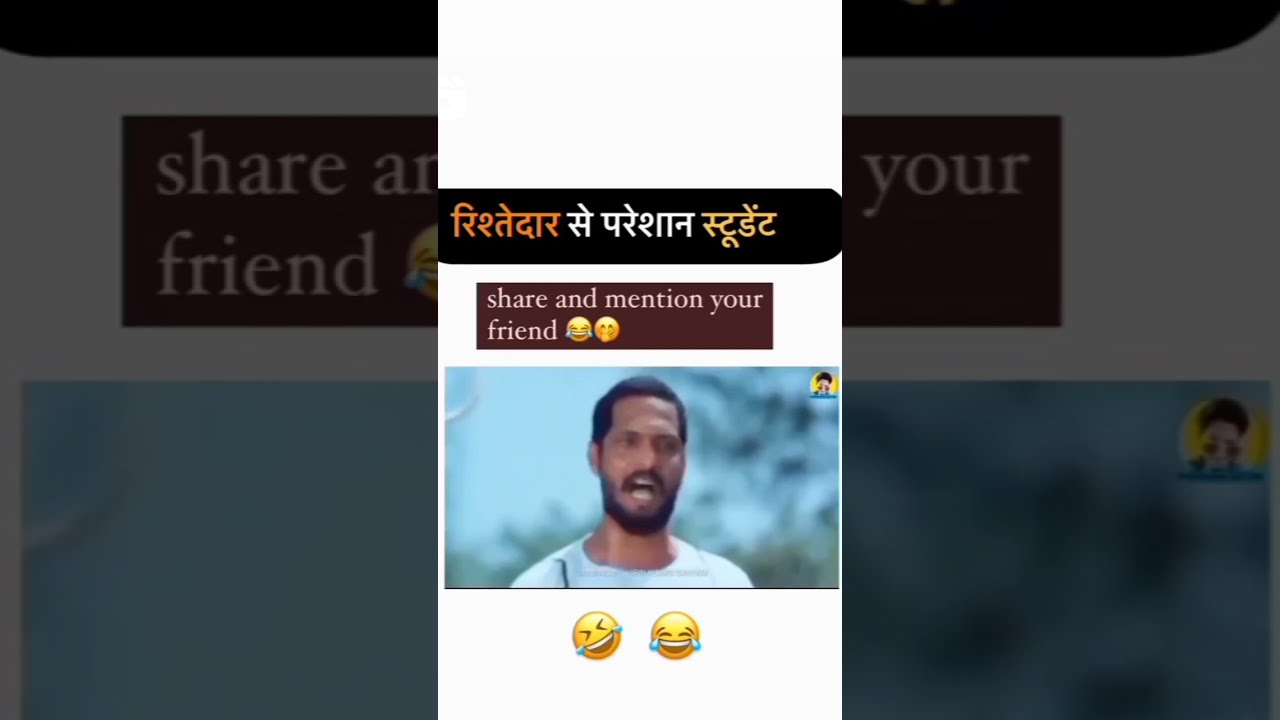The image appears to be a screenshot from an Instagram story, featuring a layered composition with a primary focus on a man standing outdoors, set against a stark white background. The man, small within the frame, has short black hair, a black mustache, and a beard. His mouth is open, giving an impression of yelling or speaking with enthusiasm or frustration. He is dressed casually in a t-shirt.

In the blurred backdrop of the image, trees can be vaguely discerned, suggesting he is outside. At the top of the image, there is a black banner with text in an unidentified language, written in orange, white, and gold font. Below this, a maroon banner displays the phrase "share and mention your friend," accompanied by a laughing emoji and an emoji with a hand covering its mouth.

Directly beneath the man's image, two laughing emojis are positioned: one tilted to the left, the other in a standard upright position. This multi-layered composition, with its various emojis and foreign text, strongly points to a social media format, likely meant to evoke humor or ridicule.